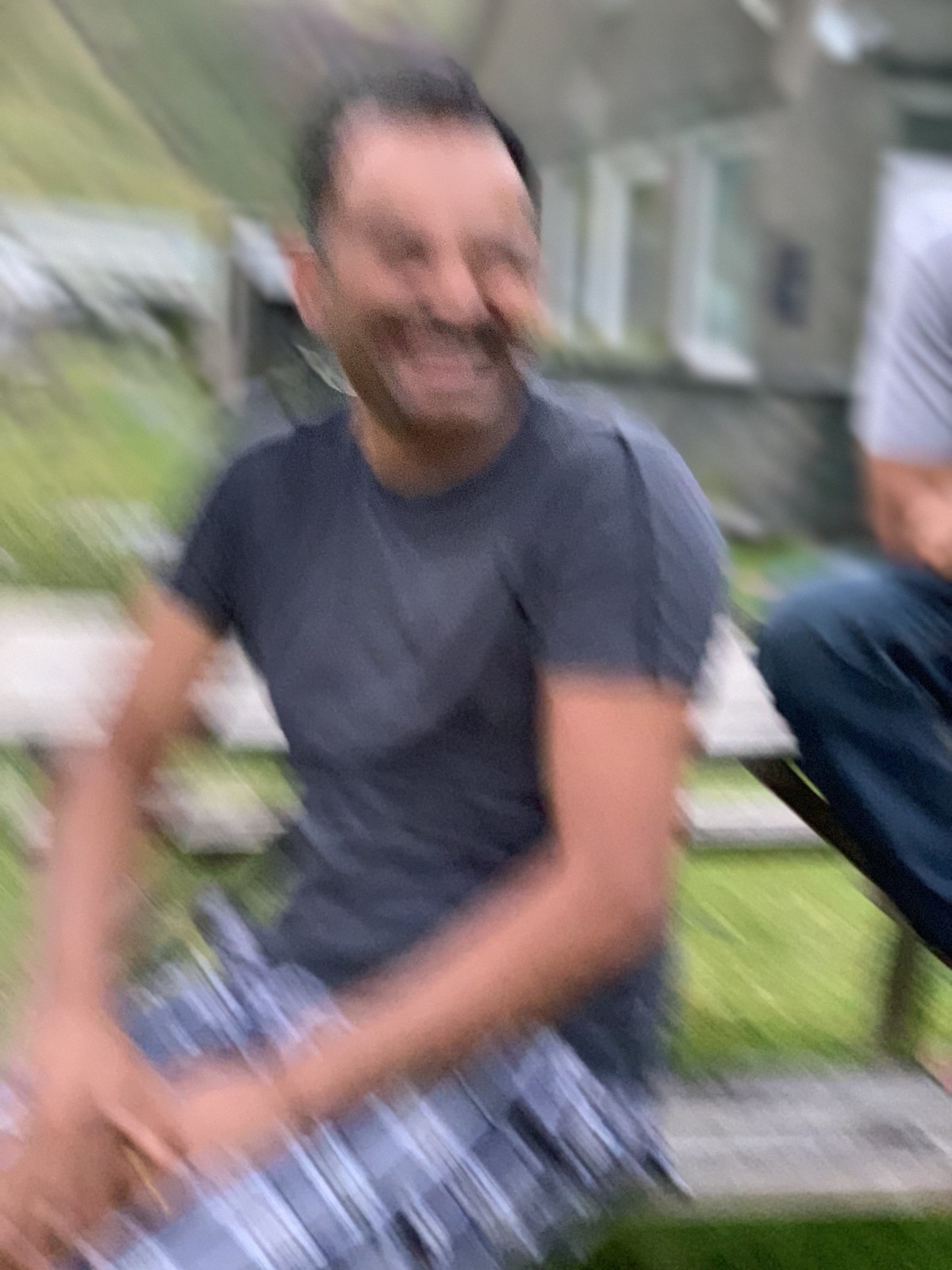The image depicts a blurry scene with visible motion blur throughout, suggesting the camera was moved while taking the picture. At the center-left of the photo, a Caucasian man sits on a gray picnic table bench. He is positioned slightly towards the left, with his body angled towards the lower left-hand corner, around a seven o'clock position, while his face is turned towards the five o'clock direction. The man is smiling, though his eyes are indistinct due to the blur. He has black short hair and some facial hair. He is dressed in a gray short-sleeved T-shirt and blue and white striped shorts. His hands rest on his lap, one layered over the other. The lower right corner of the image shows part of another person’s attire, though specific details are blurry. Surrounding the bench is green grass, and in the distant right background, a gray house with three long windows side by side is partially visible.